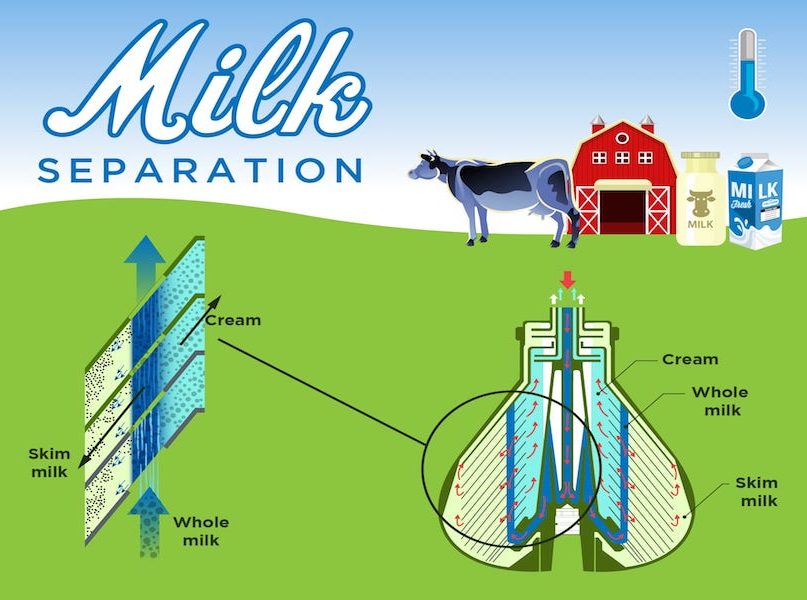The infographic is a vibrant, cartoon-style representation showcasing the process of milk separation. Set against a backdrop of a blue sky and rolling green fields, it depicts a red barn and a large cow standing prominently to the left. The title "Milk Separation" is written in blue and white at the top. Below this, the central diagram illustrates the separation process: whole milk entering from the bottom, with arrows indicating its division into skim milk (featured on the left with a white label) and cream (highlighted on the right with a lighter blue label indicating higher fat content). A thermometer to the right of the title shows that the milk needs to be chilled, with the blue mercury indicating a low temperature. Additionally, there are multiple containers of milk displayed— a glass bottle, a milk carton, and another white bottle, each adorned with the cow logo—which detail the packaging stages post-separation. Though the diagram uses arrows and color coding to explain the process, there is no supplementary text to further clarify the steps involved.